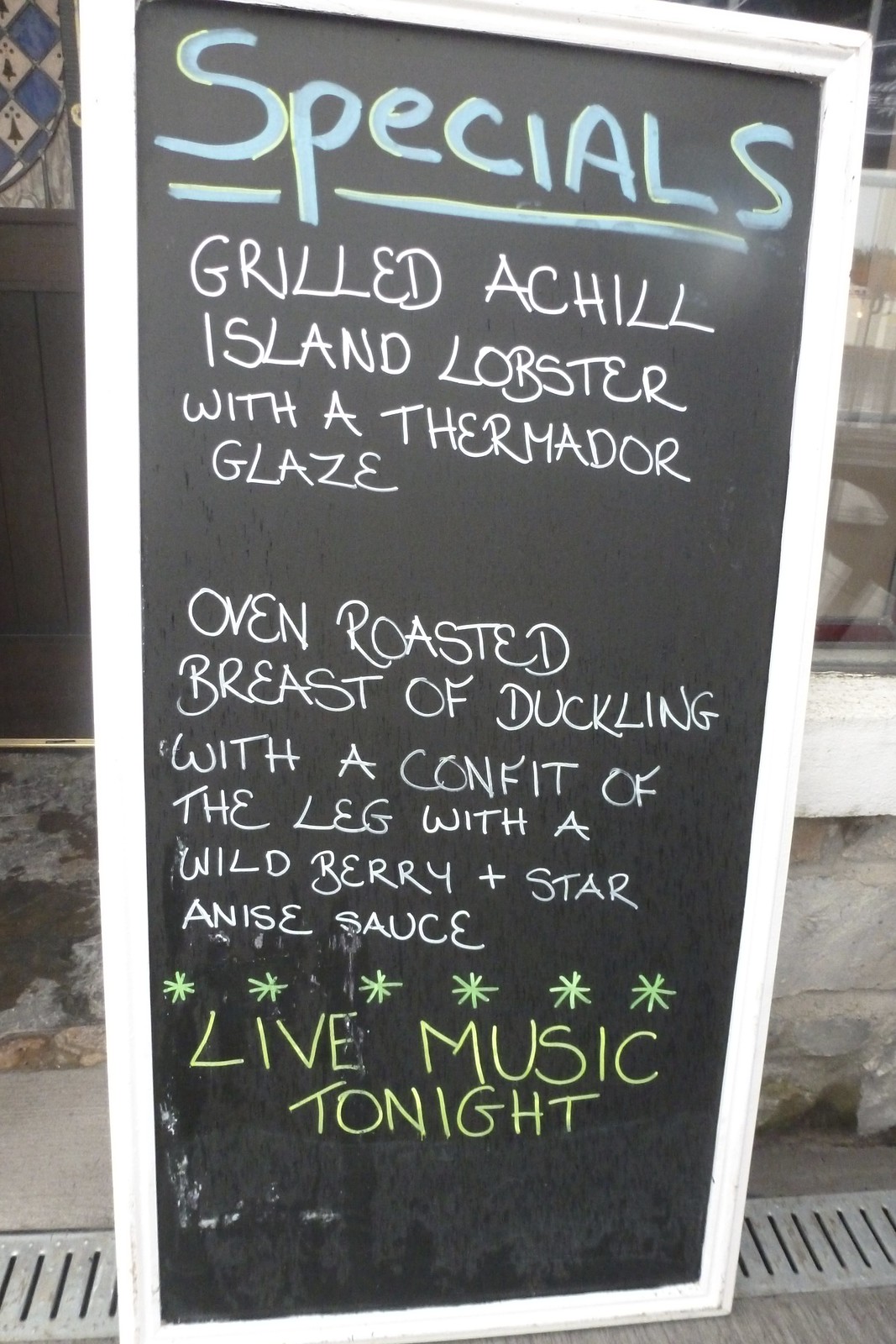This is an image of a vertical rectangular chalkboard sign outside a restaurant, framed in white wood and set against a light tan stone wall. The sign reads "Specials" at the top in light blue, underlined for emphasis. Below, in white lettering, the menu highlights "Grilled Achill, Island Lobster with a Thermador Glaze," and "Oven Roasted Breast of Duckling with a Confit of the Leg and a Wild Berry and Star Anise Sauce." Further details include six light green asterisks, and in yellow, "Live Music Tonight." The sign rests on a metal grate with horizontal slits on a gray concrete sidewalk, with a concrete block building featuring white wood trim in the background.